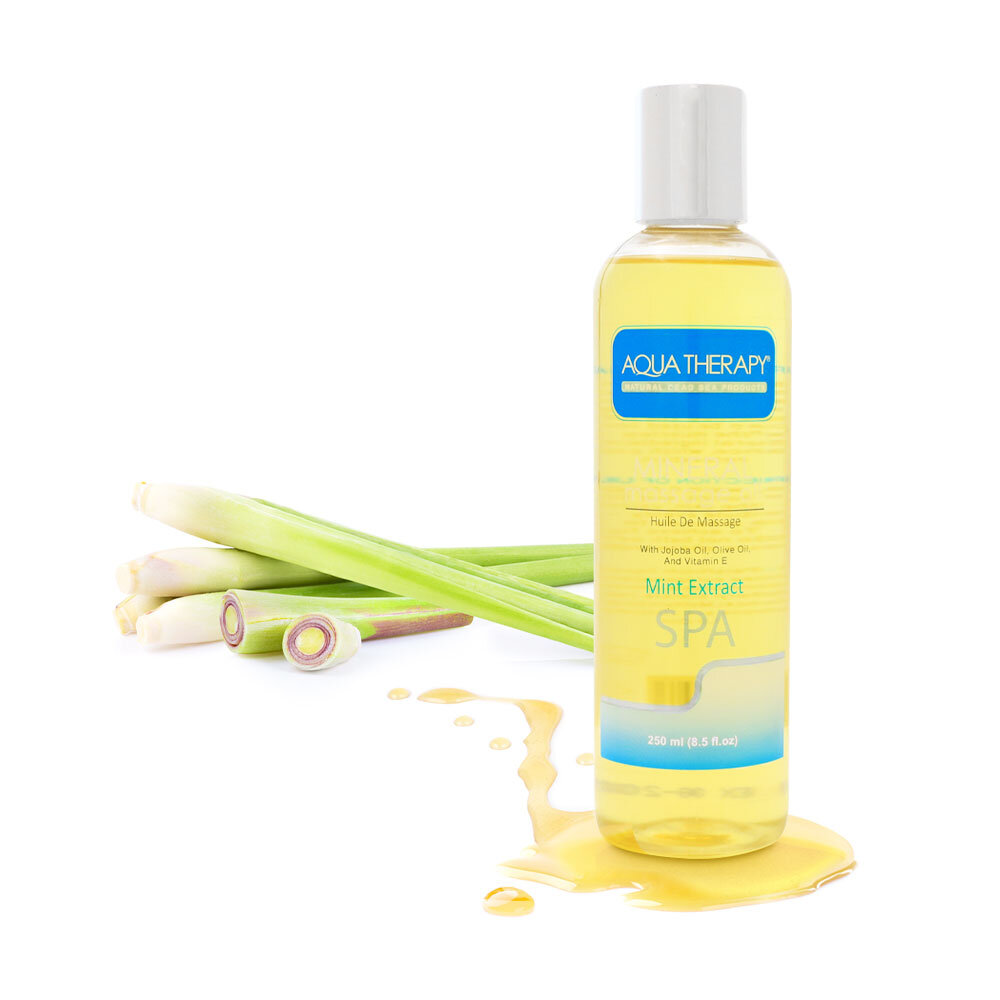The image features a tall, slender clear plastic bottle with a white cap labeled "Aqua Therapy." This product, likely a massage oil, includes ingredients such as jojoba oil, olive oil, vitamin E, and mint extract. The text on the bottle showcases words like "mint extract" and "spa" in a light green or bluish color, accompanied by the volume specifications of 250 milliliters or 8.5 fluid ounces. The oil inside the bottle is a transparent dark yellow hue. Beneath the bottle, there is a small puddle of the same oil, extending towards the background, which features some slender green stalks, possibly green onions or another type of plant that might be part of the oil's ingredients. The overall setting of the image suggests it could be part of an advertisement in a magazine or catalog, designed to showcase the product's luxurious and therapeutic qualities.